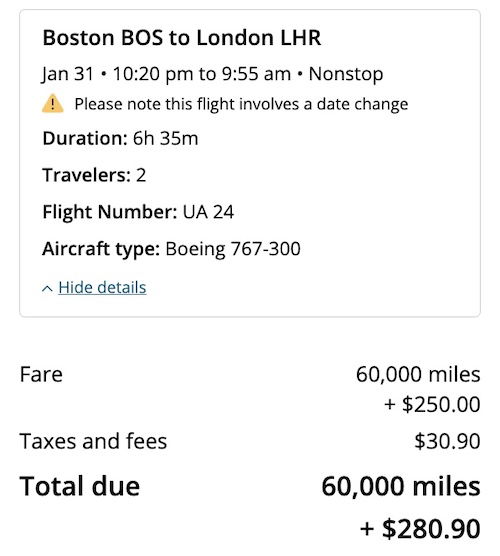Detailed Caption: 

This screenshot displays the itinerary for a non-stop flight from Boston (BOS) to London (LHR), scheduled for departure on January 31st at 10:20 p.m. and arriving on February 1st at 9:55 a.m., accounting for the date change. The flight duration is 6 hours and 35 minutes. The flight number is UA-24, operated with a Boeing 767-300 aircraft, accommodating two travelers. 

Highlighted in blue text beneath the flight details is the fare breakdown. The cost comprises 60,000 miles plus an additional $250 for the fare, along with $30.90 for taxes and fees, making the total amount due 60,000 miles and $280.90.